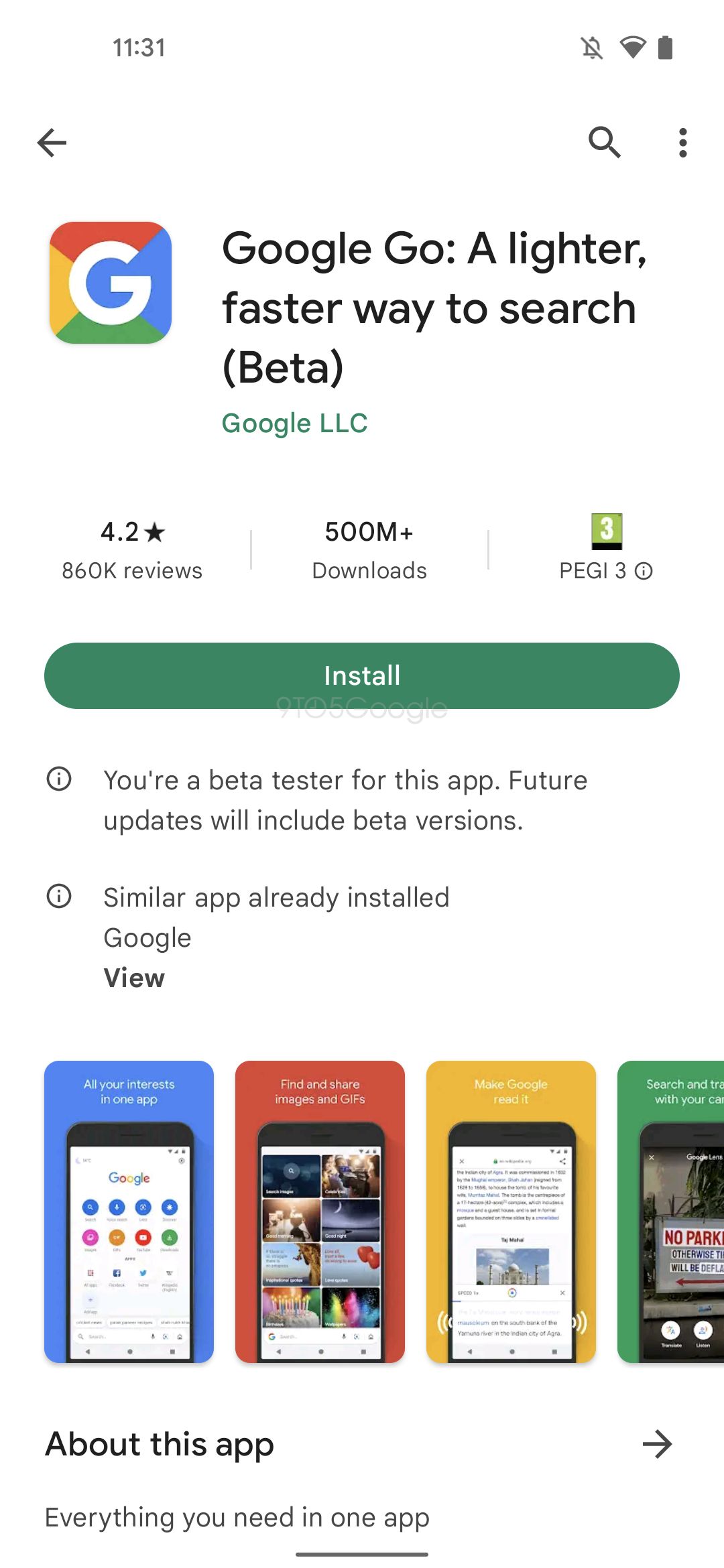The image is a screenshot captured from the Google Play app, displayed on a smartphone with a white background. 

### Top Information Bar
- **Top Left Corner:** It displays the current time, "11:31."
- **Top Right Corner:** 
  - A fully charged battery icon.
  - A Wi-Fi signal icon indicating three out of four bars.
  - A notifications icon showing that notifications are turned off.

### Navigation and Search Icons
- **Top Left Corner:** A black back arrow pointing to the left.
- **Top Right Corner:**
  - Three vertical dots symbolizing the menu options.
  - Directly to the left of the dots, there's a search icon.

### Main App Information
- **Under the Back Arrow:** 
  - A square icon with a red top, blue right side, green bottom, and yellow left side, featuring a large white "G" in the center.
  - To the right of the square, it prominently says "Google Go" in bold black text.
  - Below that, there's a lighter-text comma, followed by the phrase "A faster way to search" on the next line.
  - The word "Beta" appears on a new line.
  - Below "Beta," in green, it reads "Google LLC."
  
- **Left Side:** Includes ratings and download information.
  - **Rating:** "4.2" with a black star icon.
  - **Reviews:** "860k reviews," accompanied by a central line stating "500M+" and "Downloads."
  
- **Right Side:** 
  - A green square with a white number "3" and the label "PEGI 3" with a circle and exclamation point.
  - A long green button with the word "Install" in white.
  
### Additional Information
- **Bottom Left Section:** Two circles with an "i" inside each.
  - Two lines of information followed by a bold black "View" text beneath the lower information line.
  
- **Further Visual Elements:**
  - Multiple backgrounds in blue, red, yellow, and a partially visible green one, each with a smartphone displaying various elements.
  - Below these, in black text, it reads "About this app," paired with an arrow on the right.

- **Bottom Left Corner:** In smaller black lettering, an underlined phrase, "Everything you need in one app."